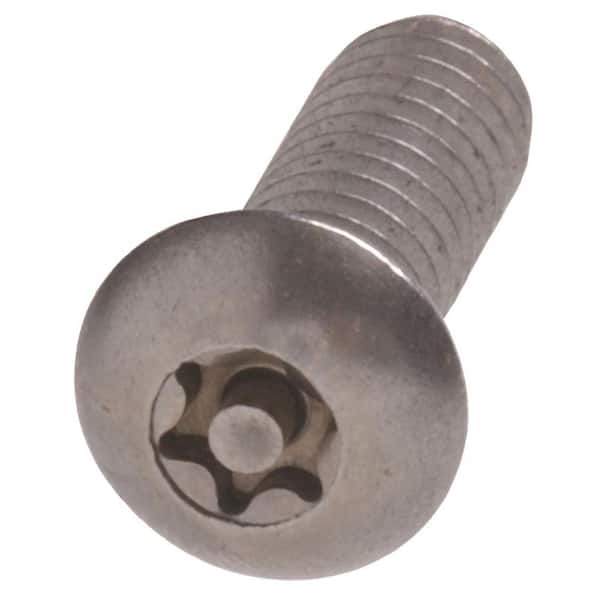The image features a single object: a specialized machine screw. The screw is centered in the photograph but slightly tilted to the right, almost creating a vertical alignment. It is silver in color, with some areas showing tarnish, especially on the threads, indicating potential prior use. The screw has a rounded top with a six-point star-shaped driver inset, which includes a small central bubble to aid in proper alignment. This specialized design and the type of threads suggest it is typically used for sheet metal applications. The close-up shot is detailed, focusing on the ridges and grooves of the screw, which show additional hints of dark gray and light brown tarnish. The photograph is set against a plain white background, emphasizing the intricate details and textures of the screw.